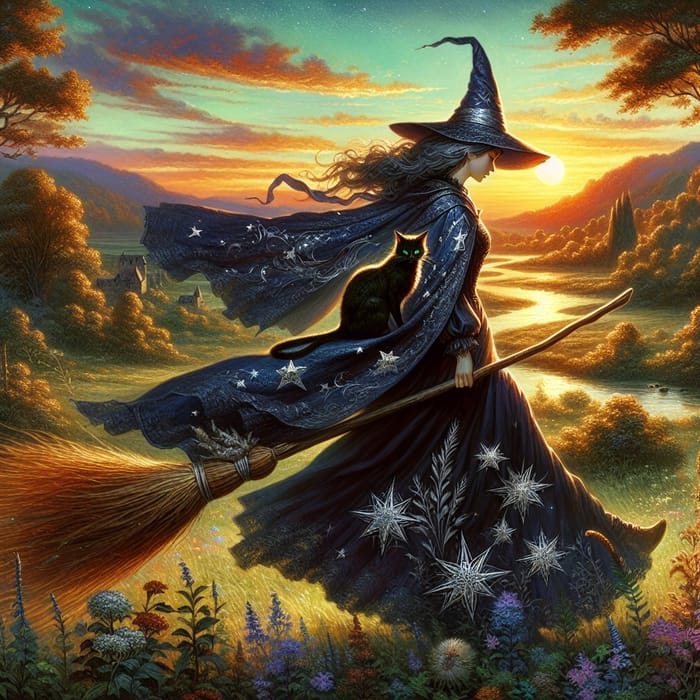This computer-generated image depicts a young, pretty witch walking through a scenic valley during sunset. The white teenage witch, with long silvery hair billowing behind her, is dressed in an elaborate dark blue robe and a pointed hat adorned with stars and other intricate embroidery. A broomstick with a crooked handle and a long, wispy end is clutched in her left hand. Perched on her billowing cape, which also has star and grass-like patterns on it, is a black cat facing the viewer, seemingly surrounded by a golden aura. 

The setting is a picturesque, flower-strewn field, with various blooms in violet, red, white, and star shapes dotting the foreground. Behind her, a stream meanders through the landscape, reflecting the light of the setting sun. The background features a mixture of trees and quaint houses to the left, with a distant castle-like structure completing the magical and serene ambiance. The witch appears to be deep in thought, looking down as she walks, immersed in the enchanting natural surroundings.